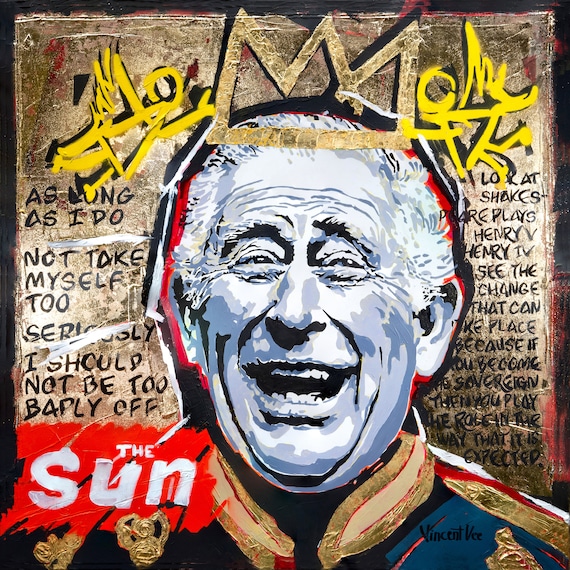The image is an artistic, graffiti-style illustration reminiscent of a special edition cover of The Sun, the British tabloid. The background features a grungy, distressed brown wood texture with some indistinct yellow graffiti. Dominating the center of the image is a satirical depiction of King Charles, dressed in a bright blue outfit and wearing a crown. He is shown with a wide, exaggerated smile, his mouth open and eyes crinkled, emphasizing a less respectful portrayal. The text surrounding him includes phrases like "As long as I do not take myself too seriously, I should not be too badly off," and references to Shakespeare's plays, such as "Henry V," "Henry IV." The entire piece, attributed to the illustrator Vincent V., seems to critique the monarchy, highlighting the changes and roles expected of a sovereign.